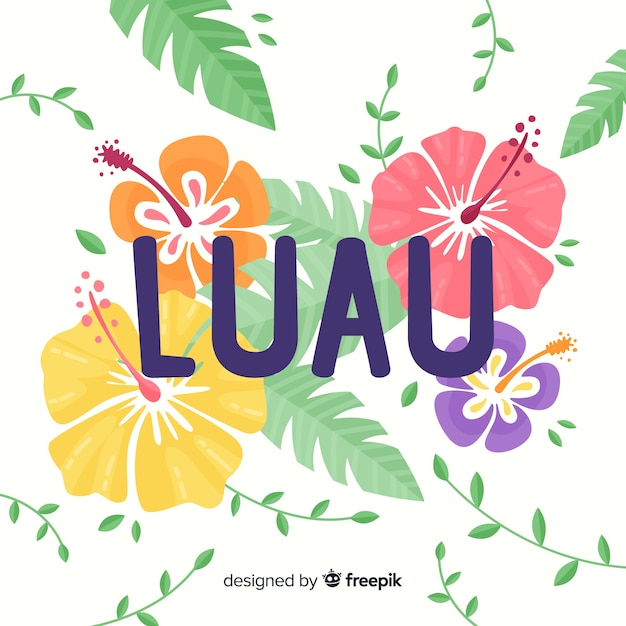The image features a vibrant Hawaiian-themed graphic design brimming with lush greenery and colorful flowers. Bright green leaves and vines, interspersed with smaller leaves, adorn the background. The centerpiece showcases four distinct Hawaiian flowers: a large yellow flower with a pink pistil, an orange flower with pink accents and a red pistil, a giant pink flower with a red pistil, and a purple flower with yellow accents and an orange pistil. These flowers are surrounded by even more green Hawaiian leaves. Dominating the center of the image, in bold capitalized dark purple letters, is the word "LU'AU." At the bottom of the image, in small black lettering, it states "designed by Freepik," with a small decorative face nestled between "designed by" and "Freepik." This visually rich composition is further adorned with small buds and offshoots in the corners, enhancing its tropical aesthetic.